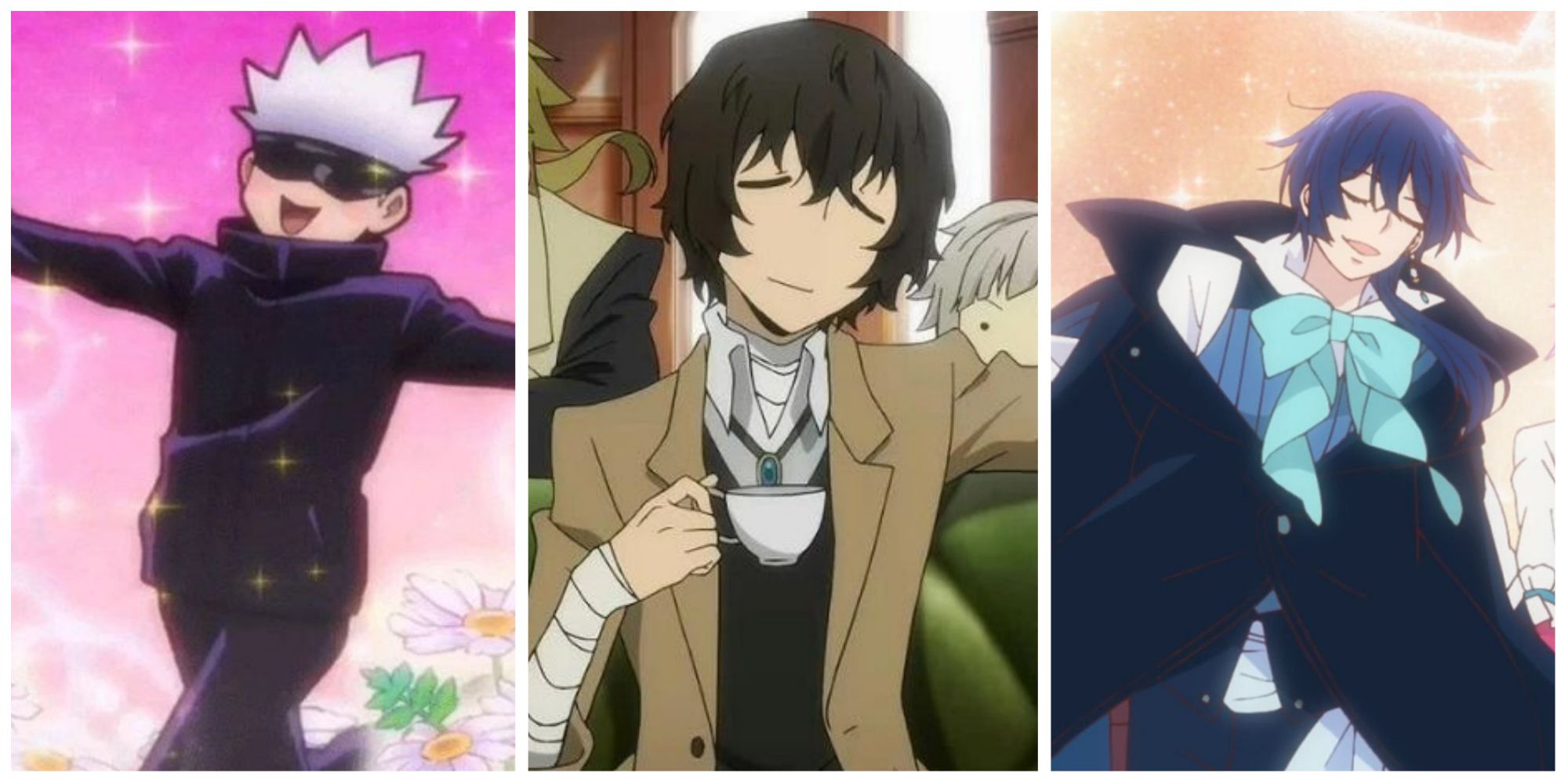The image is an anime triptych featuring three scenes of what appears to be the same character.

In the first image, the character, a young figure with spiky, white hair (or possibly a white hat) and sunglasses, is striding through a meadow of flowers against a vivid pink sky. He wears a long-sleeved, dark outfit.

The second image showcases the same character, now with short, black spiky hair and a pronounced triangular chin, dressed in a beige suit jacket. He is sitting in an Edwardian-style dining room, holding a teacup, and an emerald pendant hangs around his neck.

In the final image, the character's hair turns to a purplish-black and appears slightly longer. He sports a dark gray trench coat and a striking blue bow tie, set against a beige background, further emphasizing this character's transformation through different scenes.